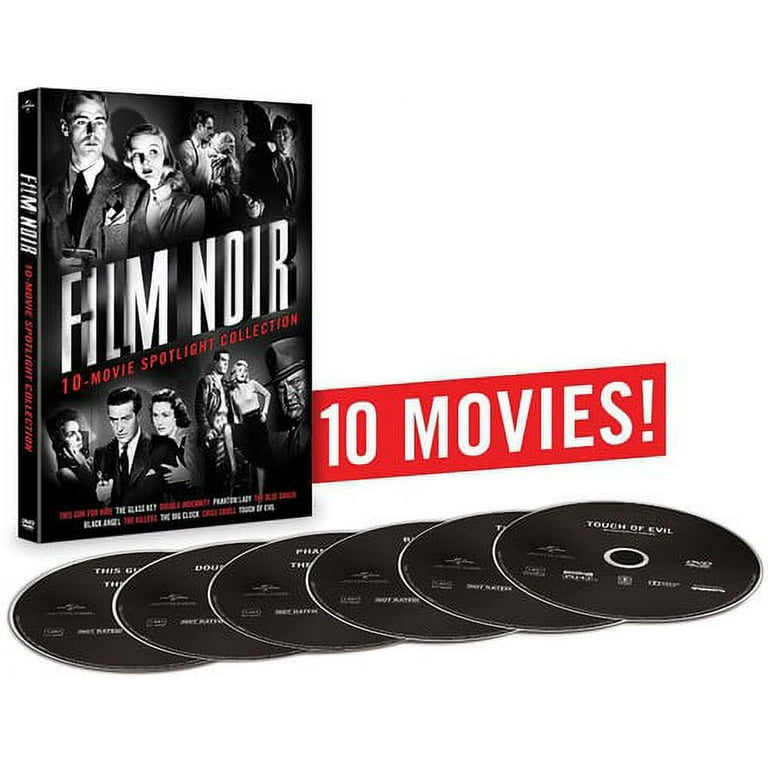The promotional image for the "Film Noir 10 Movie Spotlight Collection" prominently features a DVD case and six black circular DVDs. The DVDs are layered atop one another, with the topmost disc showing the title "Touch of Evil" in white print. The DVD case itself is depicted in black and white, showcasing various actors in classic film noir scenes: a man in a suit being held by a woman from behind, a man and a woman staring into each other's eyes, a shadowed figure in the upper right, a man holding a gun surrounded by two women in the bottom left, and two men and a woman standing together in a room in the bottom right. The text "Film Noir 10 Movie Spotlight Collection" is written both along the left-hand border and in the middle of the box. A bright red banner with white text reads "10 Movies!" on the top part of the image, enhancing the promotional appeal.